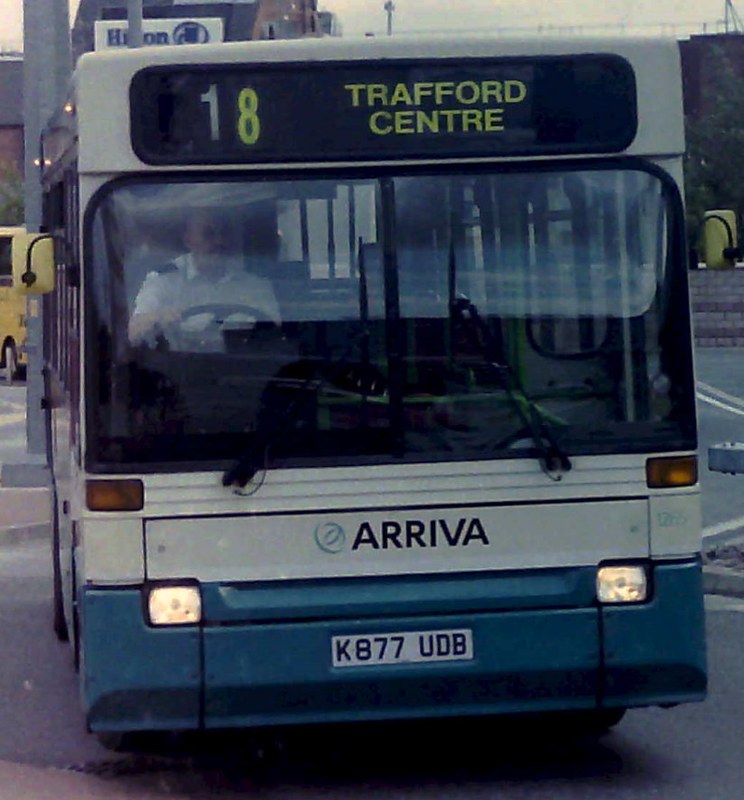This is a detailed photo capturing the front of a public bus, prominently featuring its bold elements and the surrounding urban environment. The bus takes up the majority of the frame, revealing a turquoise blue bumper and a white stripe beneath the windows. Above the large front window, the route number "18" is displayed in yellow and white, indicating the destination as "Trafford Center." The license plate is clearly visible, marked K877 UDB in black on a white background. The word "Arriva" is printed in black font on the white part of the bus below the front window. The bus driver, sporting a collared white shirt and mustache, is situated on the left side of the image, indicative of driving in a country where vehicles are right-hand drive. The scene is set in a cityscape, with faint outlines of buildings including a Hilton prominently visible in the background. Pavement and street lines are noticeable under the bus, framing the urban context of the photograph. The bus's headlights are on, and the windshield wipers are clearly seen, adding further detail to this vibrant city transit scene.